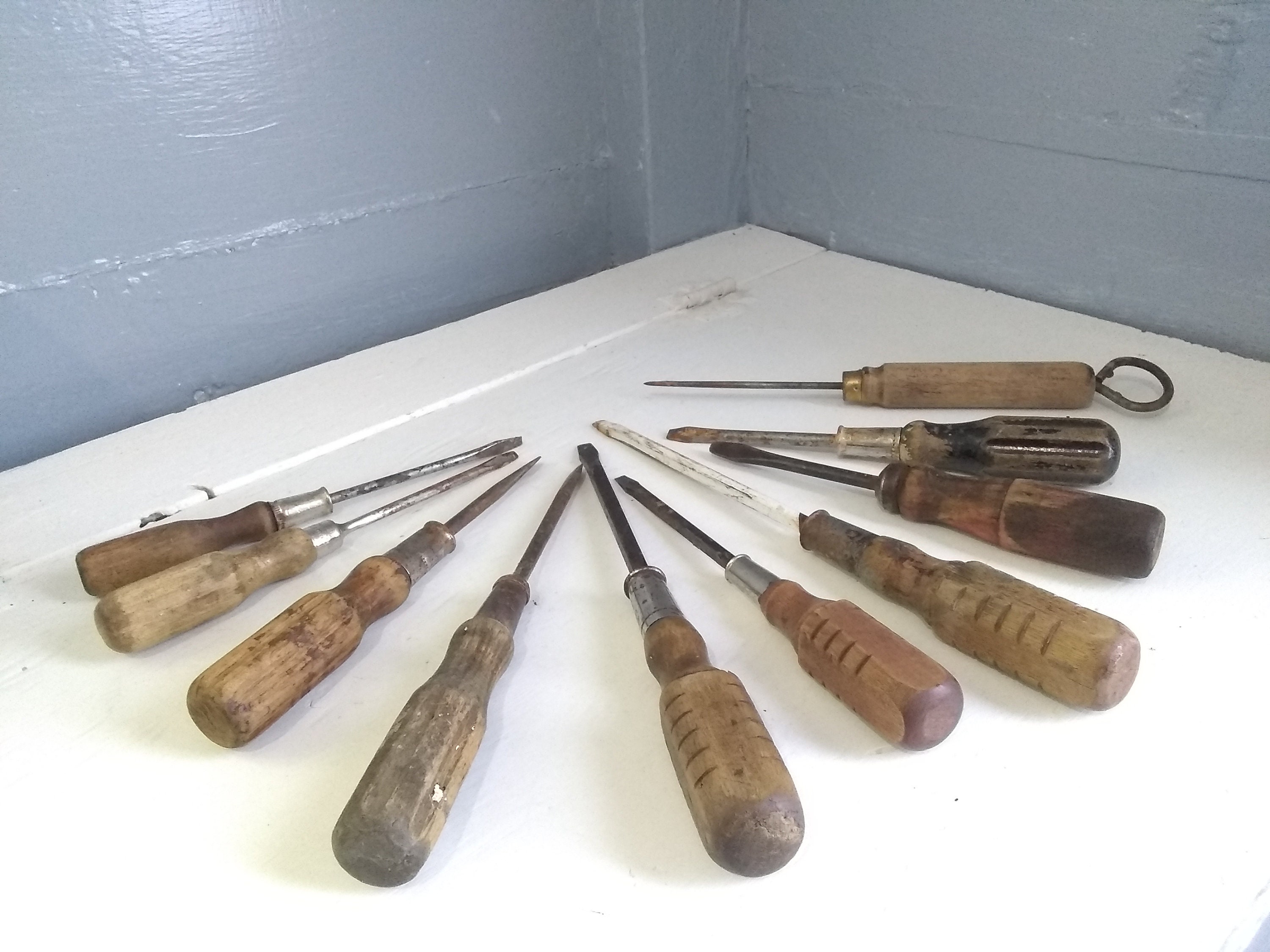The photograph captures an intriguing collection of old-fashioned screwdrivers with wooden handles, arranged meticulously in a semicircle on a crude, white-painted tabletop. The rusty, well-worn tools, some featuring metal collars and loops for hanging, are predominantly made of wood, though one may have a different handle material like plastic or resin. Among them, one tool resembles an ice pick, adding variety to the assortment. The backdrop consists of cinder block walls painted in an outdated, appealing light blue or reflective grayish-blue hue, indicating a workshop or basement setting. The focus squarely on the screwdrivers against this minimalist background brings attention to their unique, aged character.